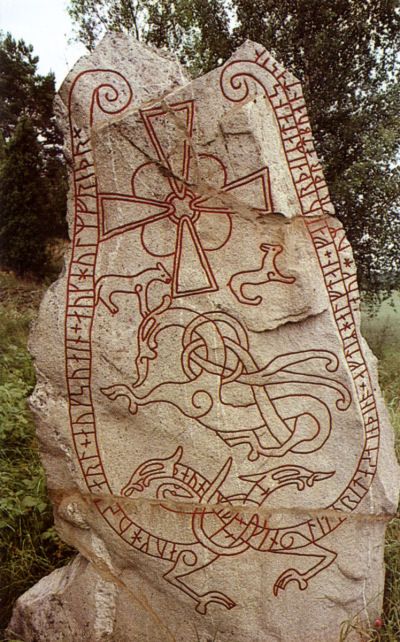The image features a large, whitish stone, prominently set in a wooded area with green trees and bushes surrounding it. The stone is intricately adorned with ancient-looking symbology that is primarily dark brown and red, suggesting an Irish or Celtic influence. Central to the stone's design is a Celtic cross-like symbol at the top center, composed of diamond-shaped or triangular elements. Flanking this symbol to the bottom left and right are animal figures, possibly representing cats, dogs, or deer. Along the sides, there are numerous letters or alphabet-like symbols intricately woven within the two dragons. The dragons' tails begin at the top and intertwine in a complex pattern before revealing their bodies crossing at the bottom. Immediately under the main cross, there is another dragon-like creature, depicted with twisty and circular lines, adding to the mystical aspect of the artwork. The entire stone stands out amidst a backdrop of green foliage and a white sky, creating a striking contrast against its natural setting.